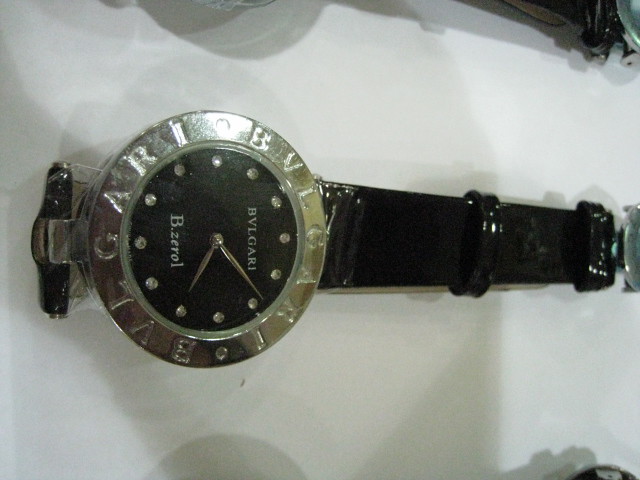This photograph showcases an elegant wristwatch with a sleek black strap and silver hardware. The watch features a sophisticated silver bezel encircling a black watch face, adorned with sparkling diamonds in place of numerals. The hands of the watch are crafted from polished silver, complementing the diamond markers. At the center of the watch face, there is white text displaying the designer’s name at the top and the model designation at the bottom, both adding to the timepiece's luxurious appeal. The bezel of the watch also carries the designer’s name etched delicately in silver. The accessory is placed on a pristine white table, with faint shadows of other objects subtly visible in the background, enhancing the overall focus on the watch’s exquisite details.